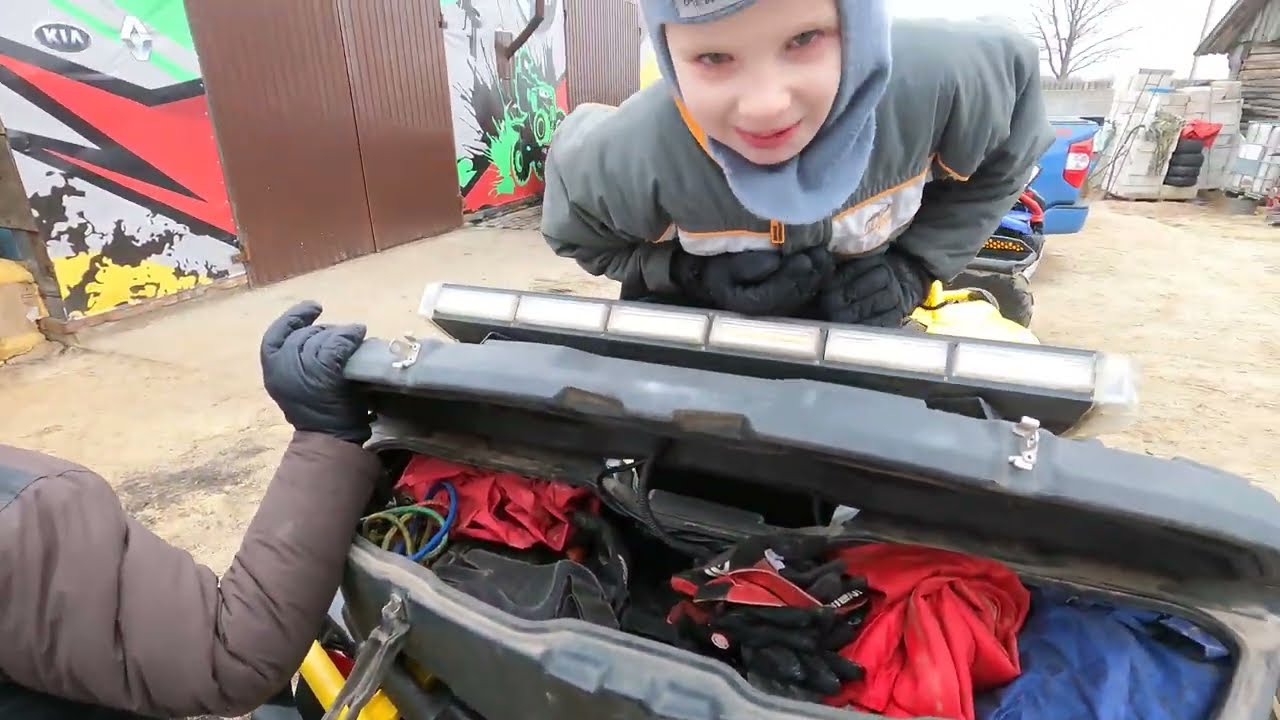The photograph captures a detailed, somewhat busy scene in a backyard setting. In the foreground, a pale-skinned child with missing eyebrows and pinkish lips is leaning over a large, heavy suitcase, which lies open to reveal an assortment of colorful clothes—blue, red, and black—and some coiled wires, with colors including blue, light blue, and yellow. The child, who appears playful, wears a blue hat, a light blue scarf around their head, and a thick gray jacket with two white chest pockets.

A person on the left, dressed in a brown puffy jacket and black gloves, holds the top left corner of the suitcase. Their face is not fully shown, but their attire suggests they are engaged in whatever activity is taking place. 

In the background, part of a pickup truck is visible along with various storage units, including stacked boxes, pieces of wood, and a brown wall adorned with two white posters featuring graffiti. This setting, along with the dirt bikes painted on the storage units, suggests a casual, potentially recreational area where the individuals might be preparing for an outdoor activity.